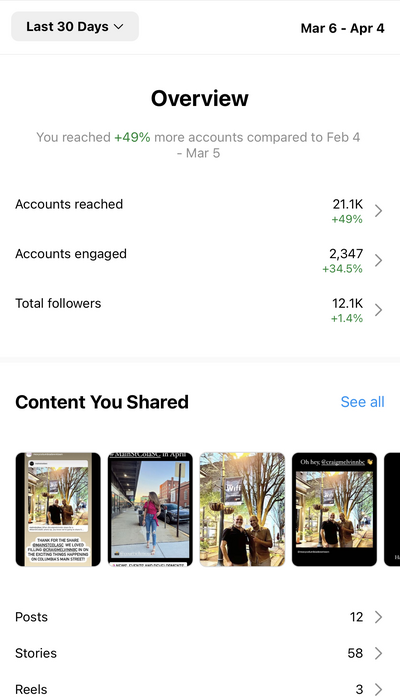The image features a detailed analytics dashboard with a predominantly white background. At the top, a thin gray line runs horizontally across the image. In the upper left corner, a light gray rectangle contains the text "Last 30 Days" in black, and beside it, the date range "MAR 6 - APR 4" (March 6th to April 4th). Below this, another thin gray line is followed by the heading "Overview" in black. Directly underneath, the text "You reach" is in gray, followed by a green "49%+" indicating a positive change. It explains that this is an increase compared to the period from February 4th to March 5th in gray text.

Continuing downward, the dashboard shows various metrics in bold black text: "Accounts Reached," "Accounts Engaged," and "Total Followers." For "Accounts Reached," the number "21.1K" is displayed in black with a "49%+" growth indicator in green below it. For "Accounts Engaged," the value "2,347" is shown in black, accompanied by a green "34.5%+" increase. Lastly, under "Total Followers," the number "12.1K" is shown in black, with a green "1.4%+" change indicated.

A thin light gray line separates this section from the rest of the image. Below this line, on the left side, there is a black label "Content You Shared" with "CEO" in blue text beside it. The section appears to depict various posts or memes, featuring images that are hard to discern when zoomed in. One set of images includes a female wearing a pink top and blue jeans. Additionally, there are three similar images of two males—one in a black shirt—smiling, with the main image being larger and the others having added text overlays.

At the bottom of the image, another black heading reads "Post Story Reels," with a value of "12.583" displayed on the right side, indicating some form of metric likely related to the shared content or engagement.

This detailed caption captures the comprehensive nature of the displayed analytics and highlights the key elements and metrics shown in the image.